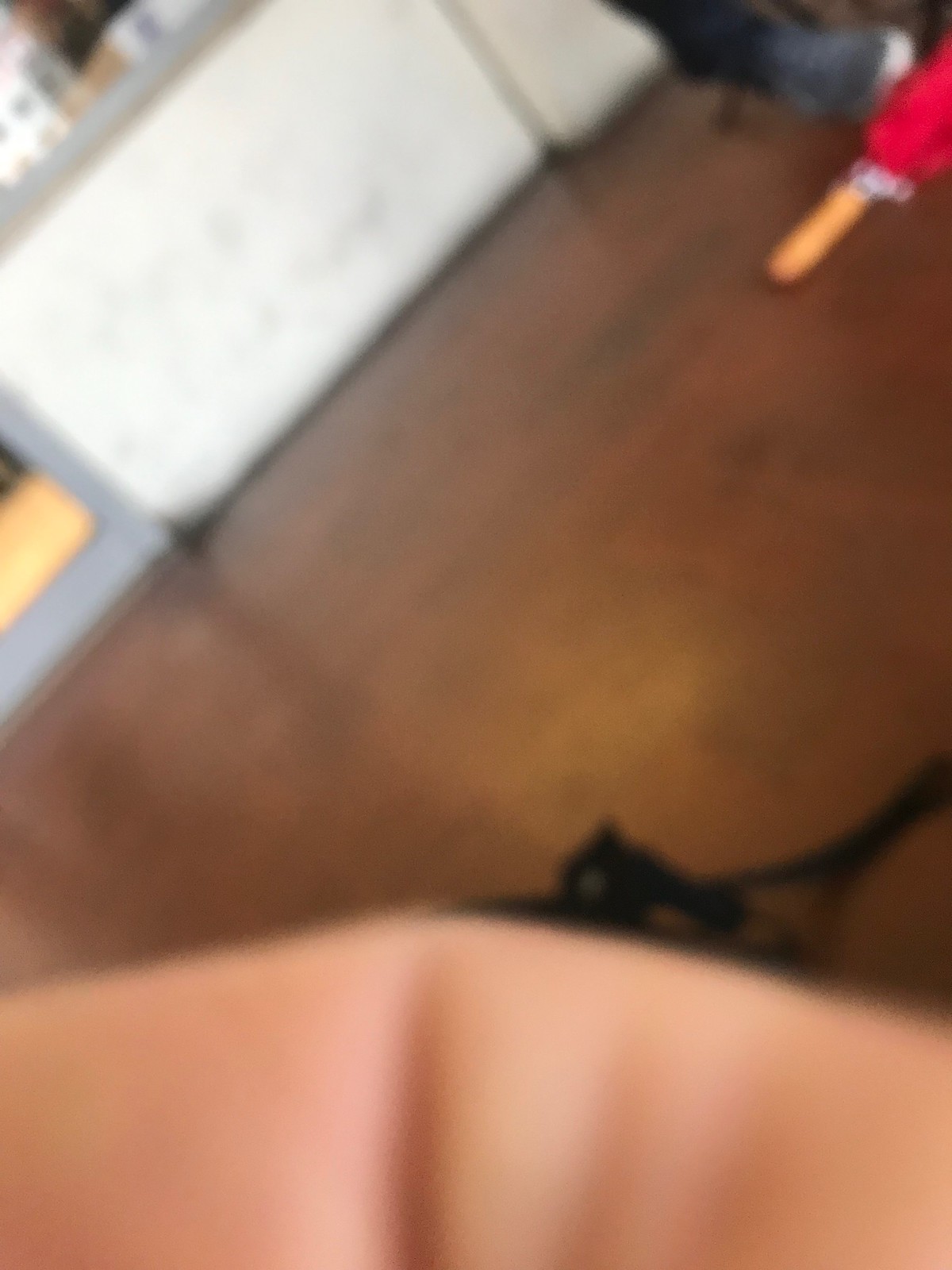The image is a very blurry and out-of-focus snapshot taken at a 45-degree angle, capturing what appears to be an indoor scene. The medium brown floor or wooden tabletop forms the majority of the background. In the foreground, there is a part of a person's finger, specifically the inside of the forefinger, which is bent, showing wrinkles at the joint near the palm. The background includes various objects: a white rectangular item trimmed in gray located towards the upper left, and a small red object with a yellow tip, possibly part of an umbrella, situated in the top part of the image. There's also what might be a lacy black undergarment on the surface. The overall composition is quite obscure due to the blurred nature of the photograph.